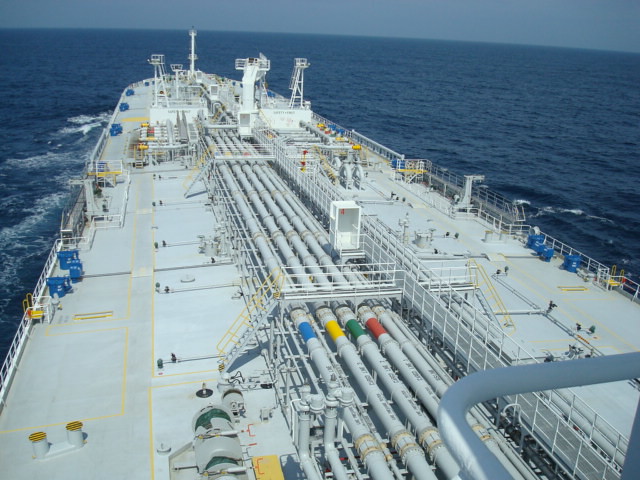This color photograph, taken in bright daylight from an elevated perspective, captures the expansive deck of a large white oil tanker sailing through a calm, deep blue ocean. The tanker is oriented toward the horizon, revealing a flat deck organized with gray pipes running longitudinally from the stern to the bow. These pipes, some adorned with blue, yellow, green, and red markings, are central to the ship's industrial purpose. The deck features walkways, with a prominent central walkway running along the ship's centerline, along with white scaffolding and perches near the bow. Additional details include railings visible at the foreground's right. No passengers are seen, emphasizing the ship’s utilitarian design. The sky is a lighter blue, merging seamlessly with the horizon, enhancing the tranquil marine setting.